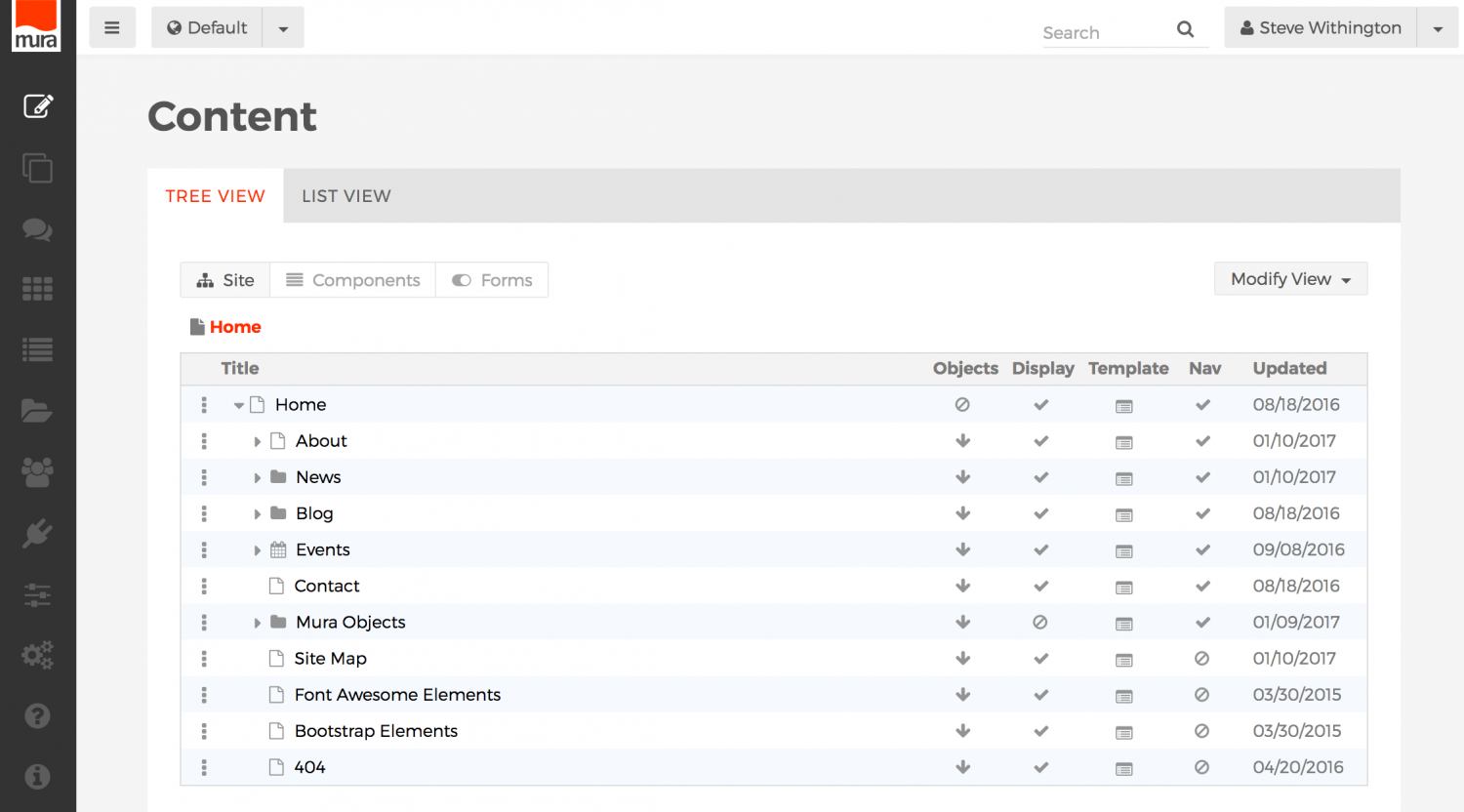Screenshot Description:

The image is a landscape-oriented screenshot from a web design or editing website, roughly twice as long as it is tall. The screenshot features several distinct sections:

1. **Left Vertical Sidebar**:
   - **Background**: Black
   - **Logo at the Top**: A white box featuring a red, wavy flag-like object with the text "Mura" (M-U-R-A).
   - **Icons Below**: Icons for editing, chat bubbles, bullet lists, files, and other functionalities.

2. **Top Horizontal Bar**:
   - **Background**: White
   - **Left Side**: 
     - Gray "hamburger" menu icon.
     - Gray drop-down rectangular box labeled "default".
   - **Right Side**:
     - White search bar.
     - Gray drop-down box with a user's name and icon labeled "Steve Whittington".

3. **Main Content Area**:
   - **Top Section**:
     - Gray box with a black header labeled "Content".
     - Inside this gray box:
       - White tab with orange text labeled "Tree View" (highlighted).
       - Long rectangular gray box labeled "List View" with black text.

   - **Middle Section**:
     - Options labeled "Sites", "Components", and "Forms".

   - **Bottom Section**:
     - Orange header labeled "Home".
     - List of files in a staggered order with various displayed options.

This detailed breakdown accurately describes the layout and elements contained in the screenshot, providing a clear understanding of its structure.